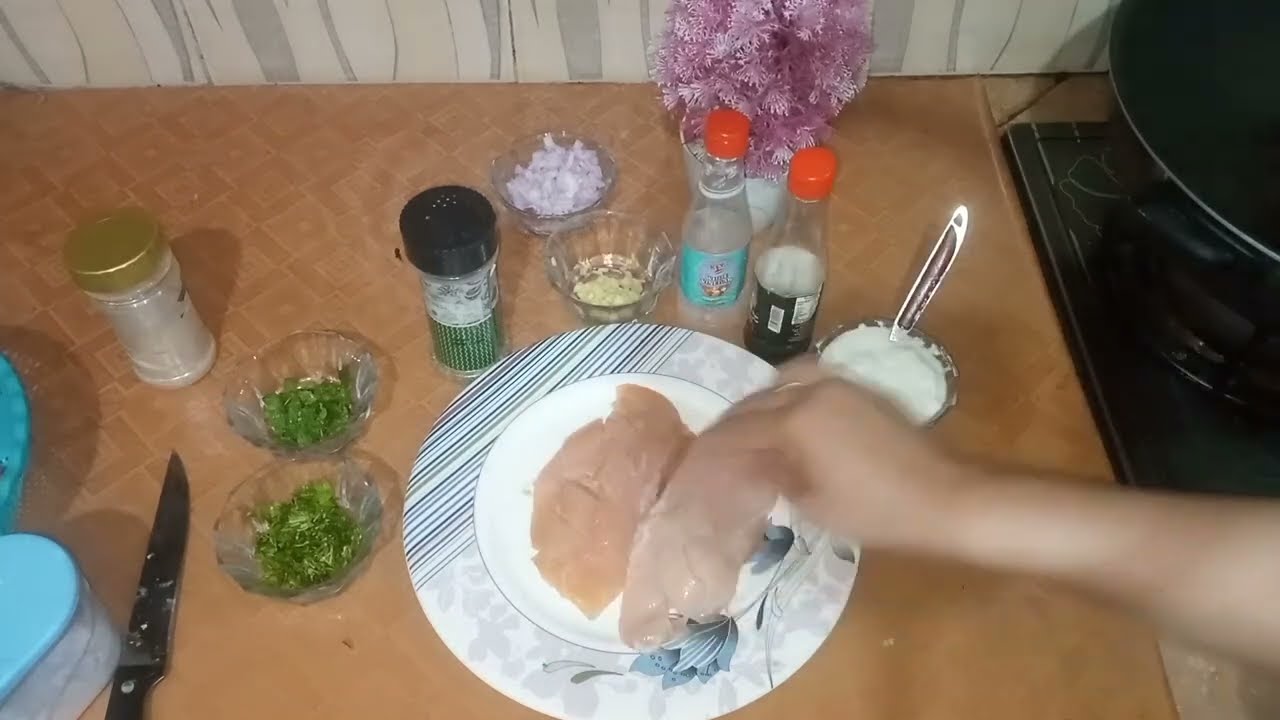In this first-person perspective still from a Facebook cooking short video, the focus is on a white plate adorned with an intricate floral border featuring blue and gray flowers. Central to the plate are two raw chicken breasts, their pale tan color and irregular shapes clearly visible. A hand emerges from the lower right corner, grasping one of the chicken breasts. Surrounding the plate is a meticulous arrangement of small glass bowls containing various green herbs and chopped onions, as well as a mixture that appears to be garlic. Additionally, there are two spice bottles—one with a black lid and the other with a gold lid—as well as a couple of nearly empty plastic bottles with red lids, possibly containing sauces or condiments. Positioned on a brown countertop, this preparation scene also includes a clear container holding a white, mayonnaise-like substance and a knife in the bottom left corner. On the right side of the image, a stove with a skillet indicates the next phase of cooking is imminent, completing this detailed setup of a culinary endeavor preparing to transform raw ingredients into a savory meal.